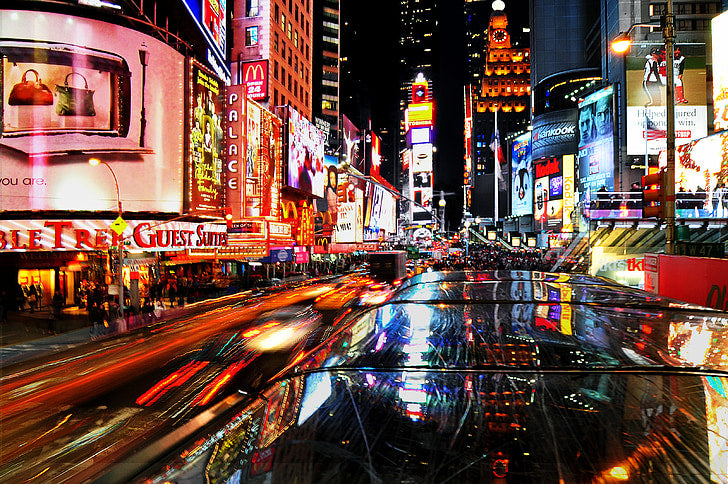A vibrant time-lapse photograph captures the bustling nightlife of a busy city metropolis, likely New York City's iconic Times Square. The image showcases cars speeding down a main thoroughfare, their lights leaving bright, colorful trails against the dark night. The sidewalks teem with numerous people, adding to the energy of the scene. From the perspective behind a vehicle in the foreground, the Doubletree Hotel prominently stands on the left, accompanied by a neighboring sign that reads "Palace." Further down the left side of the street, a McDonald’s and other businesses illuminate the night with neon signs. The right side is equally lively, featuring a street lamp and numerous neon billboards, including advertisements for a prize fight and an animated film characterized by a glowing penguin. A large building crowned with a tall clock tower and additional neon billboards adds to the grandeur of the cityscape. A ticket booth on the right side of the thoroughfare solidifies the location as Times Square, reflecting the vibrant, nonstop energy of this famous New York City landmark.